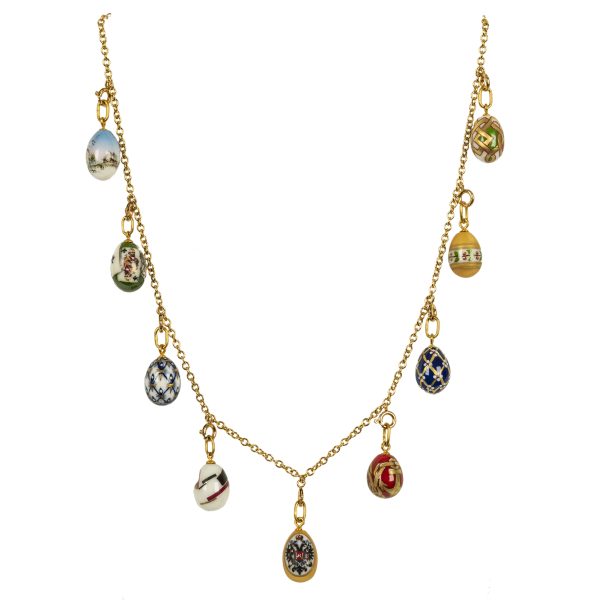The image features a delicate gold necklace set against a stark white background, giving it a floating appearance. The thin chain-link necklace forms a gentle 'V' shape and is adorned symmetrically with nine egg-shaped pendants, each boasting unique designs and colors. Starting from the top left, the pendants showcase a variety of patterns: one with a blue and white motif reminiscent of a serene sky, followed by a green charm featuring a playing card design, then another blue and white pendant. Next is an intricate design with blue, white, and brown elements, while the central bottom pendant displays a gold, blue, and red crest-like pattern. Ascending the right side, there's a red and gold pendant, a blue one with gold accents, a yellow pendant with a central band, and finally, a gold, green, and white-striped charm. The minimalist background and absence of any additional elements keep the focus squarely on the necklace and its artfully designed pendants.